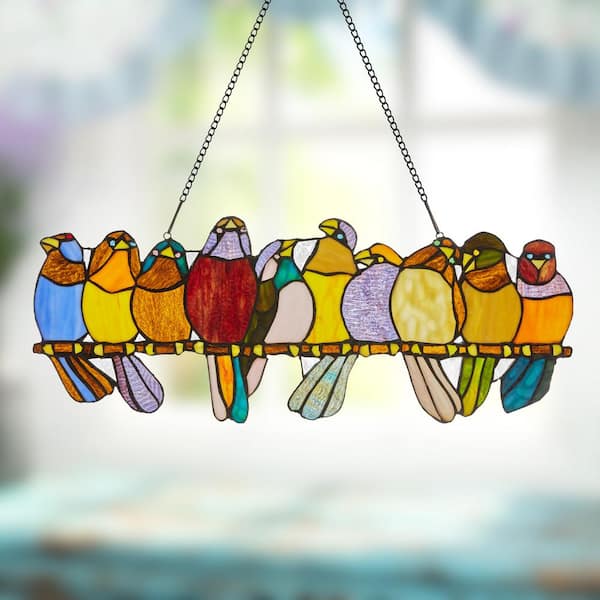This photograph captures a vibrant stained glass ornament that hangs from two black metal chains in a window, with a blurred background highlighting its intricate details. The centerpiece of the ornament features ten beautifully crafted birds perching side by side on a stained glass branch adorned with varying shades of brown and yellow. Each bird, viewed from the front, boasts a unique palette and position, enhancing the overall charm. The array includes birds in blue, golden yellow, bright yellow, brass-like hues, wine-red, multicolored shades with brown wings and green and white breasts, pastel purple, light brown, and orange. Some birds tilt slightly, while two at the center gaze at each other, adding a sense of interaction amidst the colorful array. Their vivid yellow beaks contrast strikingly with their diverse plumage, reminiscent of Goldfinches and Robins but presented in imaginative, non-representative colors.